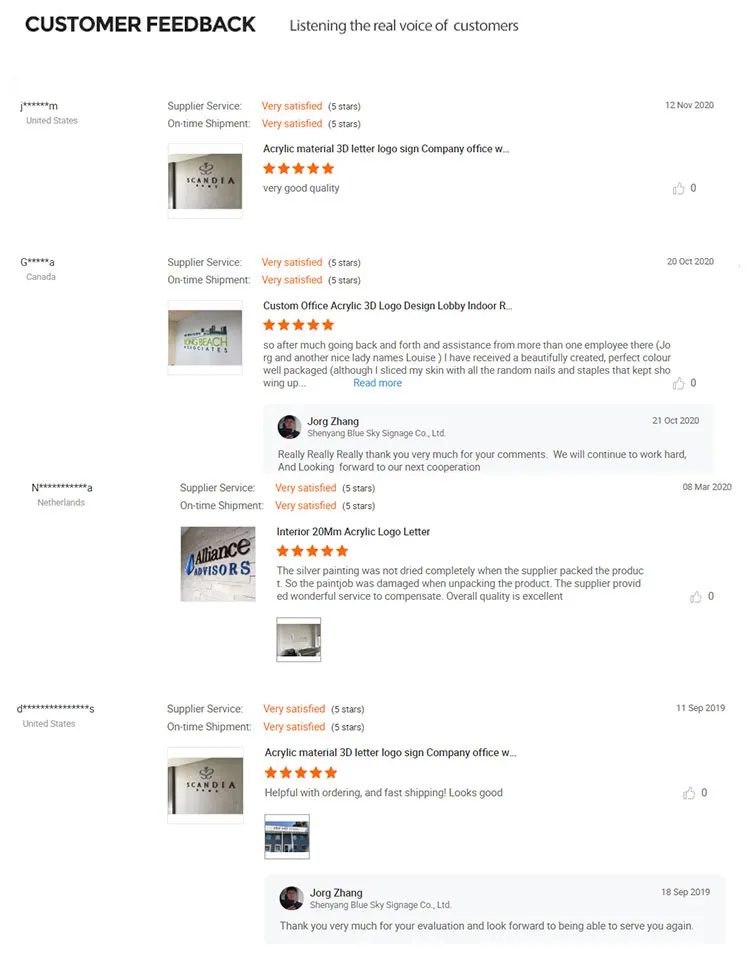The image depicts a webpage with a white background, giving the appearance of an edge-less design. Dominating the top-left corner, bold black text reads "CUSTOMER FEEDBACK." To its right, in smaller black font, the phrase "Listening, The Real Voice of Customers" is displayed. 

Below this header, a series of reviews are presented. Each review starts with a username followed by "United States," and is indented slightly to the right with details about the review. The first review mentions "Supplier Service" rated as "Very Satisfied" with five orange stars. This is followed by "On-Time Shipment," also rated "Very Satisfied" with five orange stars.

Further below, there is an image of a silver-colored appliance, though the specific details are difficult to discern. Accompanying this image, the text reads "Acrylic Material, 3D Letter Logo, Sign Company, Office, W..." Below this description, five orange stars are displayed, accompanied by the text "Very Good Quality."

This pattern is repeated for three more reviews, each following the same format and spanning a quarter of the page in a vertical layout.